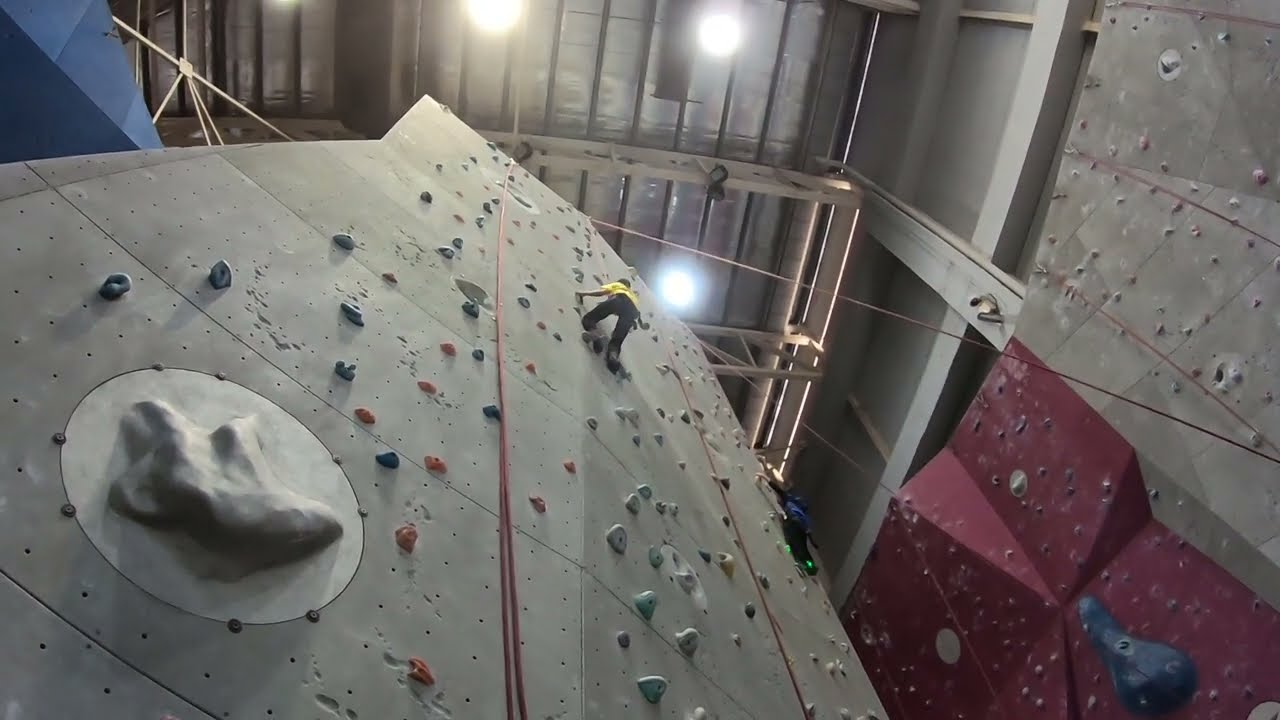This photograph captures an indoor rock climbing facility from a ground-level perspective, looking up at two climbers making their way up separate walls. Centered in the image is a climber dressed in a yellow top and black pants, ascending a gray concrete climbing wall lined with variously colored handholds, predominantly gray, with some red and blue ones interspersed. The wall is equipped with numerous spaces for hand and foot placement, essential for navigating the climb. Overhead, bright white or yellow circular lights illuminate the scene, and the ceiling is partially visible, adding to the sense of height. To the right of the main wall, another climbing wall comes into view; this one features a more complex design with inclines and sections that jut out, suggesting an advanced level of difficulty. A second climber, attired in a blue shirt and black pants, can be seen partway up this adjacent wall. The overall setting appears to be indoors, with a blend of gray, white, blue, maroon, and black colors contributing to the atmosphere. There are no visible texts or signs in the image.